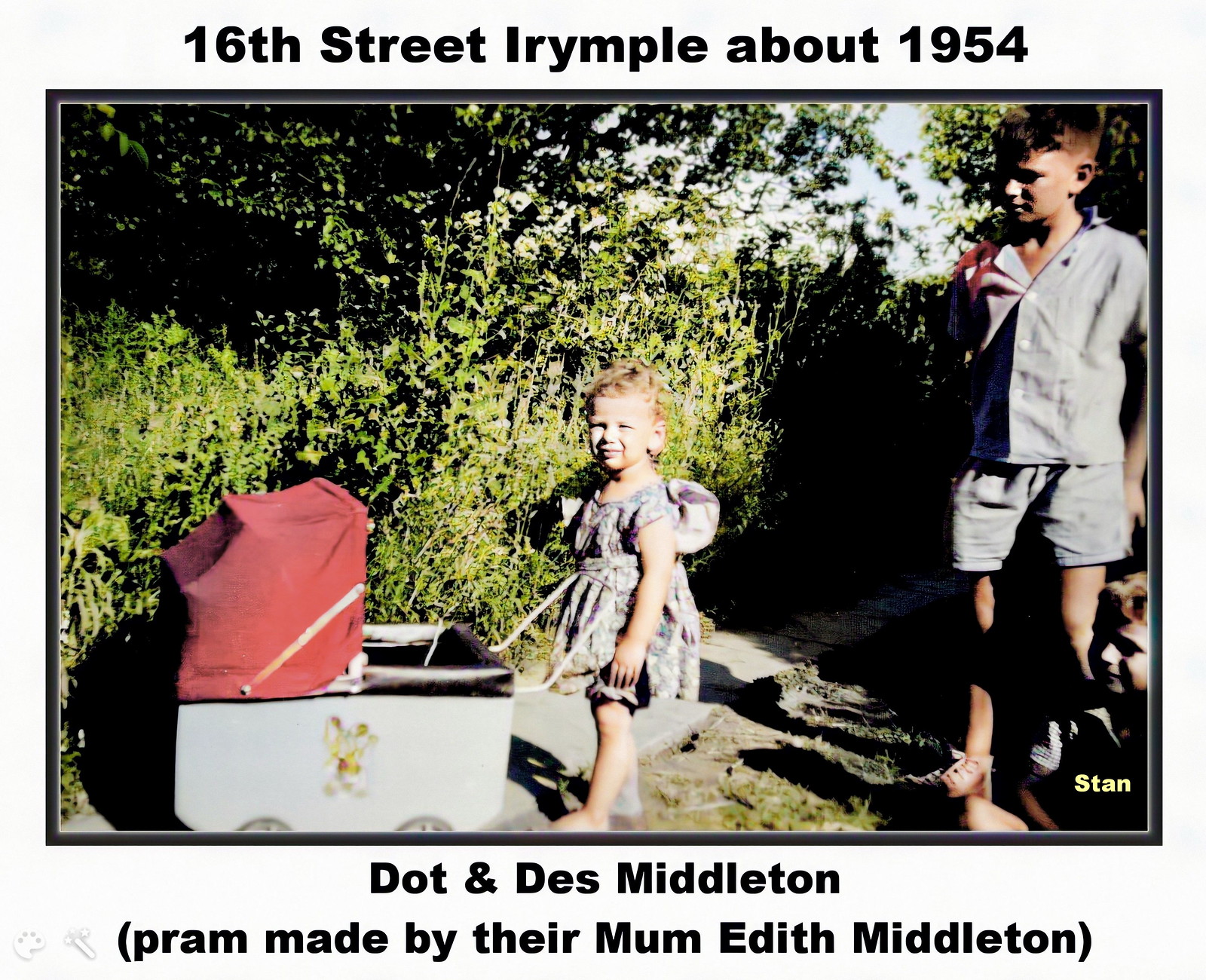A horizontally aligned rectangular photo from 1954 titled "16th Street, Irymple" features two children, Dot and Des Middleton, standing in front of a pram made by their mother, Edith Middleton. The photograph has a light gray background and is bordered by  a dark gray border. The pram, an old-fashioned white stroller with a red top and a blurry frontal decoration, stands on the grass and dirt.

To the right of the pram, a little barefoot girl wearing a floral pattern dress with ruffled sleeves stands, likely around two years old. She has short, curly blonde hair. Next to her is a boy, around 10 years old, in shorts and a button-down shirt, with short brown hair looking down at her. Partially visible in the lower right-hand corner is another child, a boy named Stan, sitting on the grass, with part of his body obscured by the edge of the image and his name printed in yellow letters. In the background, there's a blue sky visible in the upper right-hand corner. Along the left side of the photo runs a little gray walkway bordered by large weeds or bushes.